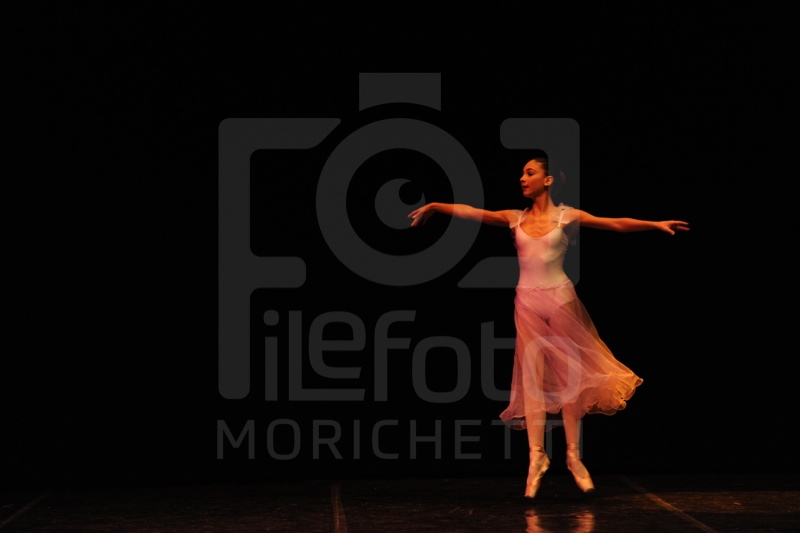In this detailed and captivating image, we see a female dancer in her 20s, prominently illuminated against a darker, solid black background, creating a striking contrast. The image is of landscape orientation and captures her in a dynamic pose, mid-dance, with her arms fully extended to both sides. She stands slightly to the right of the center of the frame, looking to her left in profile. 

Her attire consists of a sleeveless white blouse paired with a lacy, transparent pink overskirt that elegantly falls just below her knees. She’s poised on her toes in white ballet slippers, either slightly off the floor or just touching it, with her reflection faintly visible on the dark surface beneath her.

Behind her, a large sign dominates the backdrop in big, bold white letters, reading "F-I-L-E-F-O-T-O," with a large circular O above the text, possibly forming part of a logo or watermark effect. Below this text, additional letters "M-O-R-I-C-H-E-T-T" are visible, adding to the graphic elements of the photo. The image, with its blend of representational realism and artistic flair, perfectly captures the grace and poise of the dancer amidst a minimalist yet impactful setting.